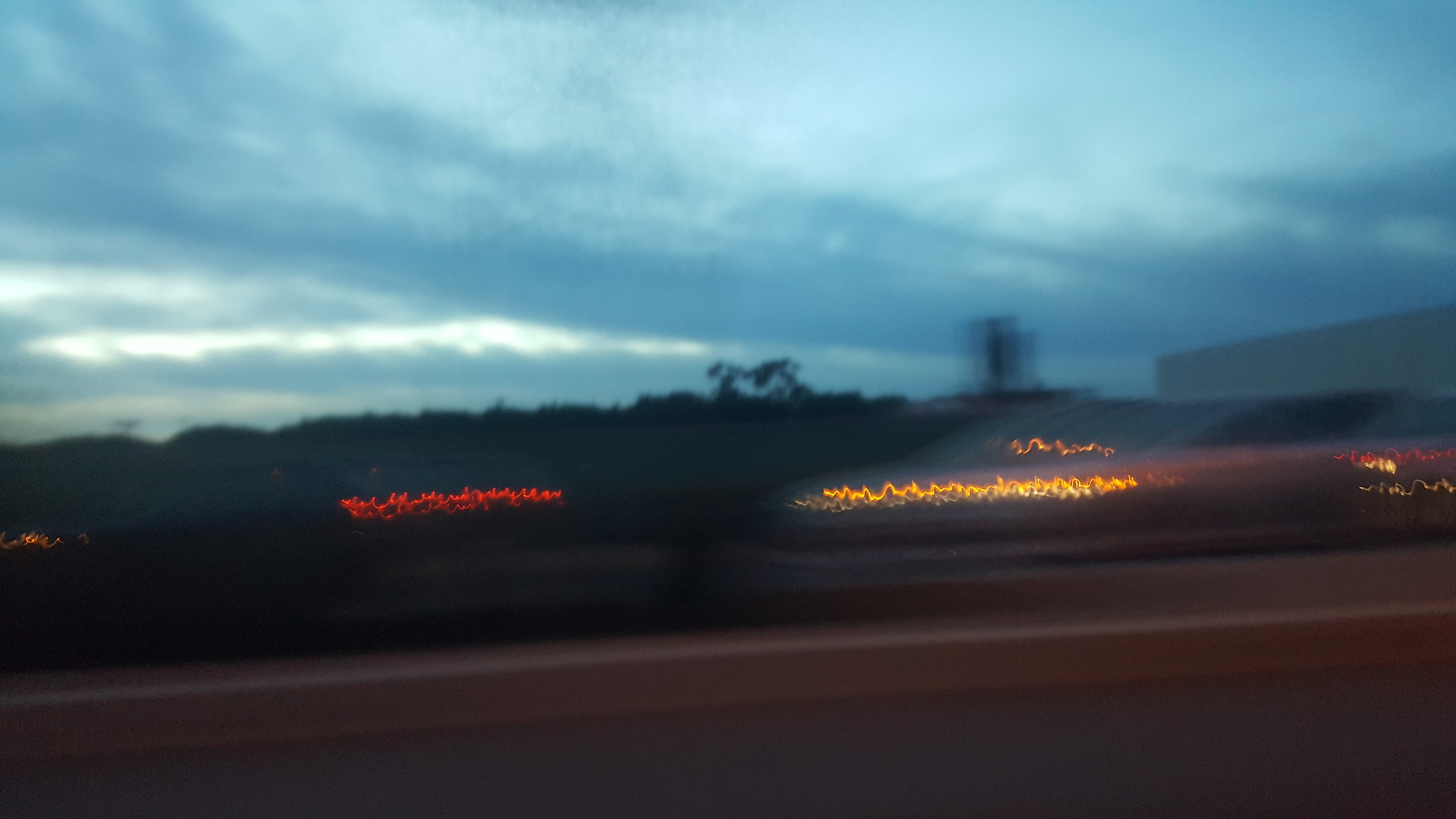A blurry nighttime photograph captures the view from inside a moving car, looking across a guardrail at oncoming traffic. The dark, cloud-filled sky creates a moody backdrop, while a distant tree line marks the horizon. Directly across from the moving car, a silver or beige sedan travels in the opposite direction, its headlights and side lights transformed into wavy, golden lines due to the motion blur. These light trails, along with similar red squiggly lines in the background, add an abstract quality to the image. The scene is enveloped in darkness, with the squiggly lines of light providing the only sources of illumination, creating an almost surreal, otherworldly atmosphere.